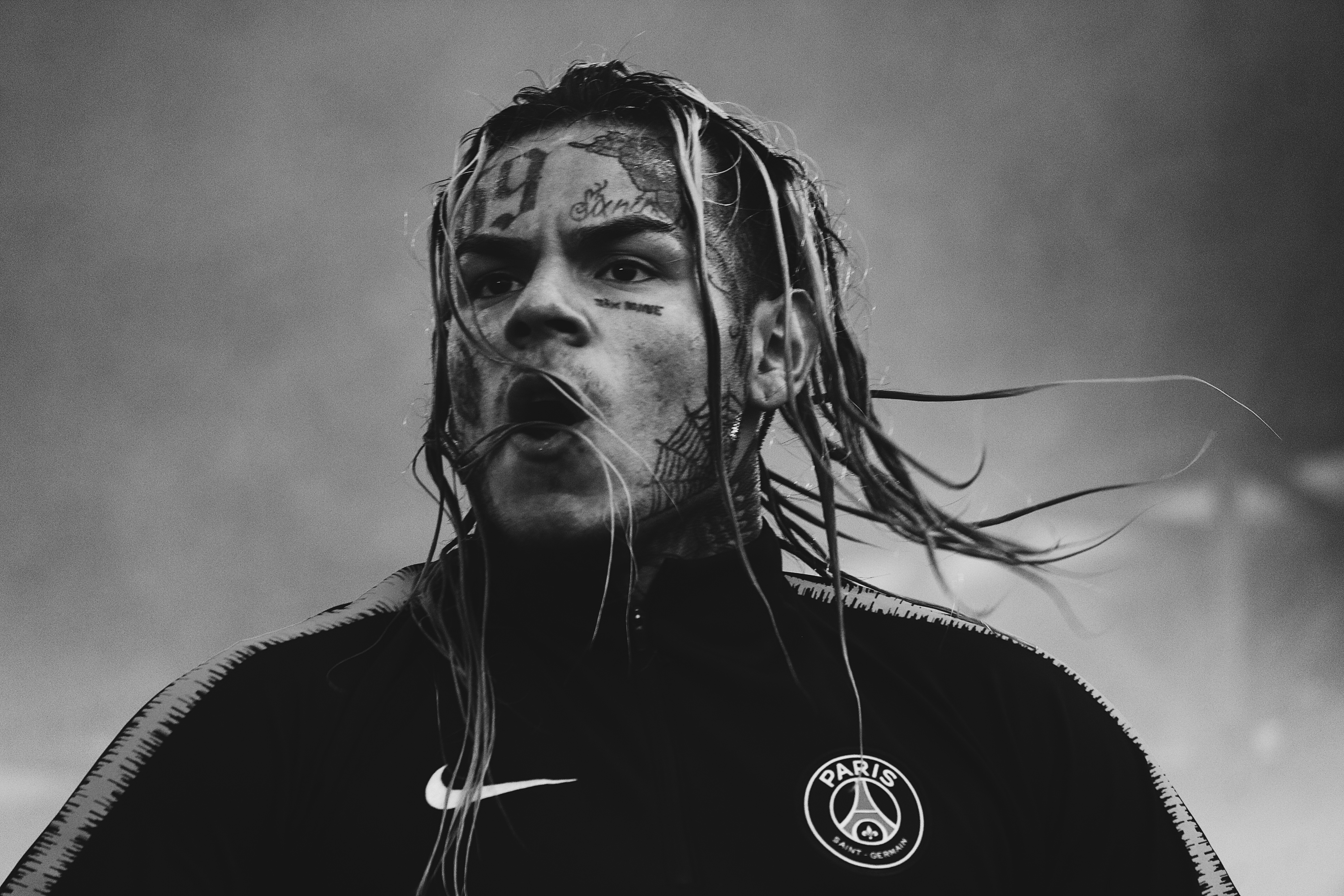The black-and-white photograph features a young man centered against a completely gray background, giving an impression of an overcast or foggy day. He appears to be in his 20s, with pale skin and straggly long hair that reaches his shoulders, blowing slightly in the wind. The man is dressed in a dark-colored Nike athletic jacket, adorned with white stripes along the sides and a Nike swoosh on the right side of his chest. Additionally, he sports a circular logo on his jacket's left shoulder, featuring an illustration of the Eiffel Tower with "Paris" inscribed above it.

The most striking features of the man are his numerous facial tattoos. Prominently, he has a large "69" tattoo on his forehead, a spiderweb tattoo extending from beneath his ear to his neck, and various other designs scattered across his face. These include a rose partially concealed by his hair on the upper left side of his forehead, lettering tattoos above and below his left eye, and additional markings on his cheeks. The man is looking slightly to the left, giving the image a sense of depth and introspection. Without any other objects or text in the image, the focus remains entirely on the man and his detailed appearance, highlighted starkly in the monochromatic palette.